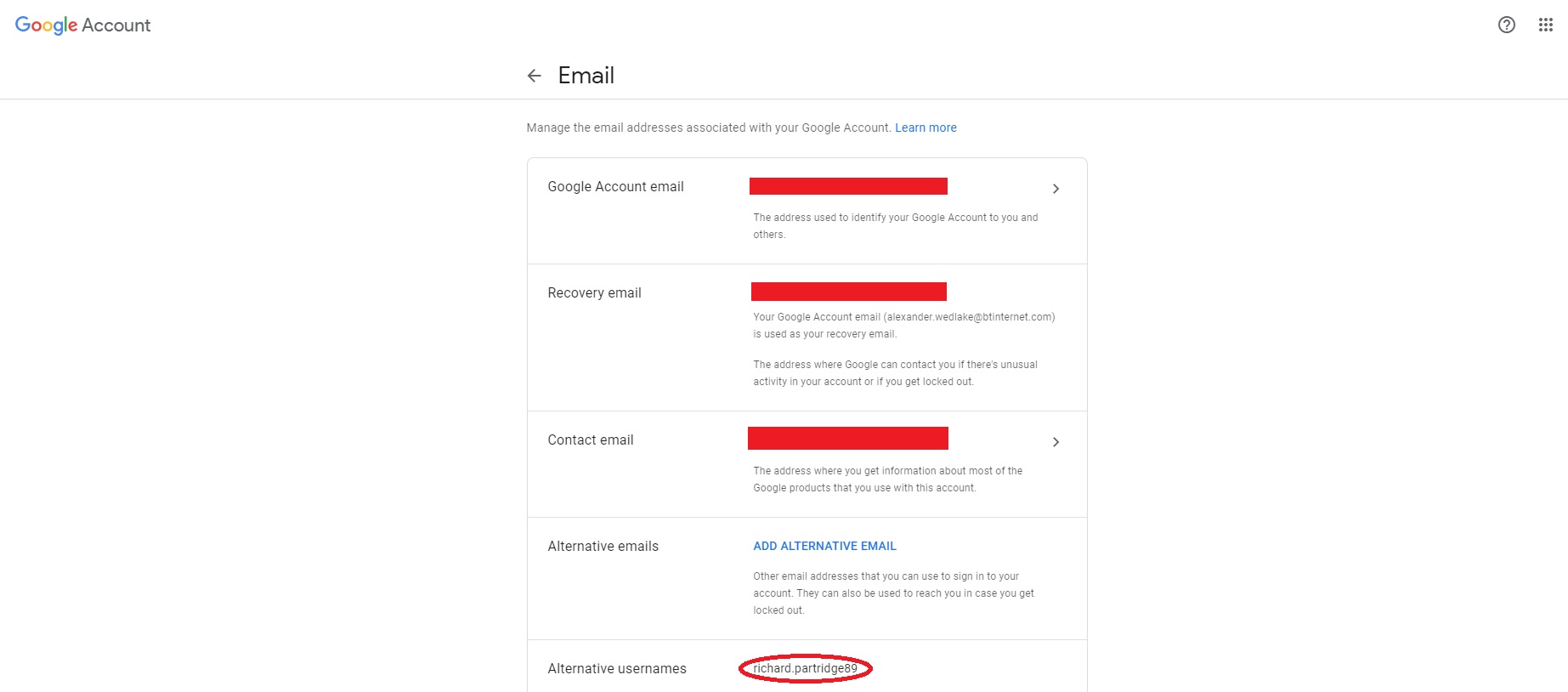This image is a screenshot from the Google account settings page on a desktop or laptop computer. The design is minimalistic with a plain white background. In the top-left corner, the word "Google" is displayed in its signature colored letters: blue, red, yellow, blue, green, and red. Directly next to it, the word "Account" is written in black. 

In the top-right corner, there is an icon of a question mark inside a circle, which users can click to get help. Next to this is the 'nine-dot' grid icon, often referred to as the app launcher or 'Google Apps menu,' which opens a panel of Google services.

Centrally featured on the page, the heading "Email" appears with a back arrow icon beside it. Below this heading, it says, "Manage the email addresses associated with your Google Account," followed by a "Learn more" link that is clickable for additional information.

The section under "Google account email" highlighted with a red bar, explains, "The address used to identify your Google account to you and others." Following this, the "Recovery email" section clarifies that your Google account email also serves as the recovery email, used for contact if there’s unusual activity or if you get locked out. The next section, labeled "Contact email," designates the address where you receive information about most of the Google products you use with the account.

Towards the bottom, there is a section for "Alternative emails," accompanied by a blue link that reads "Add alternative email." At the very bottom of the page is the "Alternative usernames" section, which includes the user’s alternative username, "Richard.partridge89," circled in red.